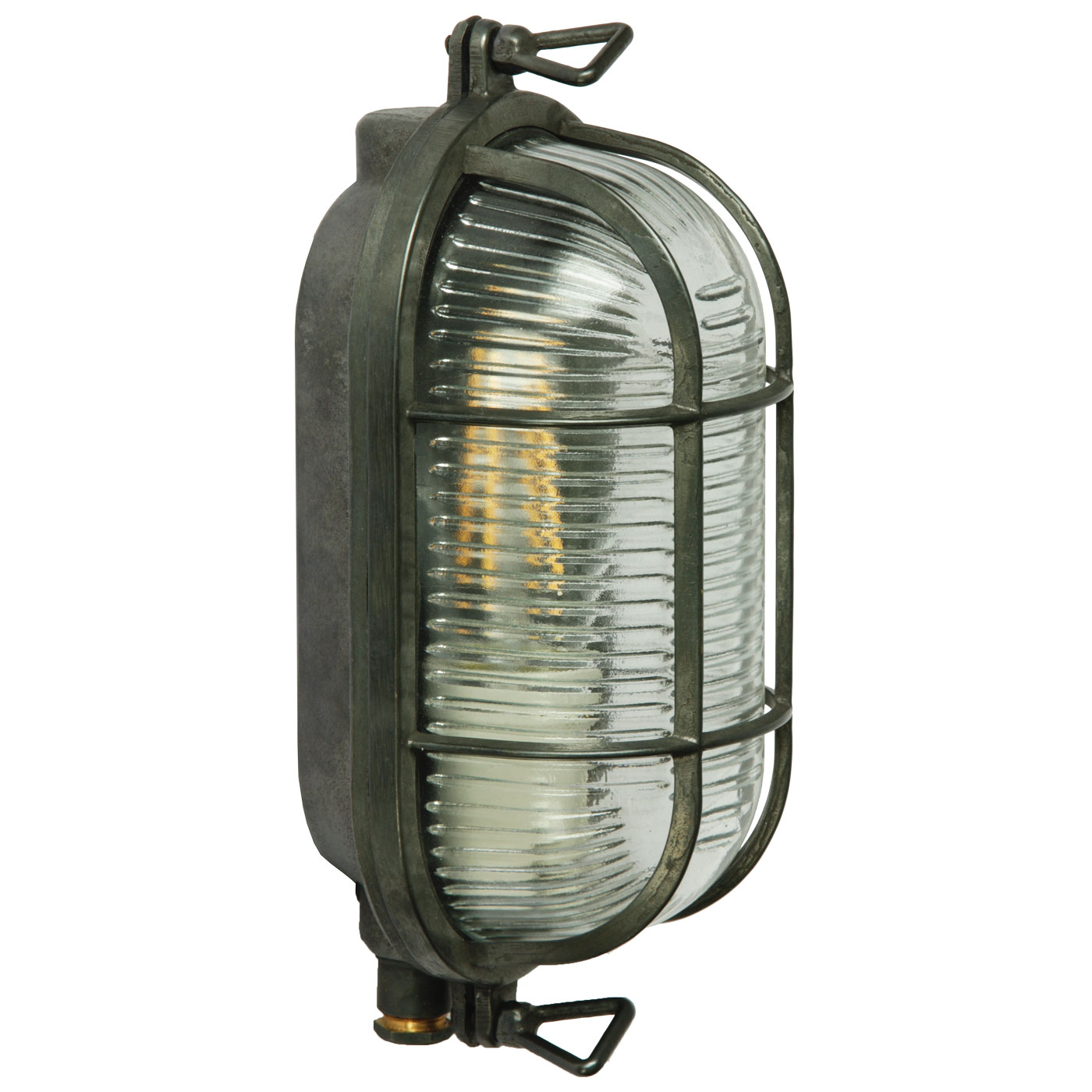The image features a vintage-style outdoor lantern lamp in a dark charcoal gray or blackish color, viewed from an angle that shows both the side and a portion of the front. The lamp has a frosted glass front with horizontal grooves, obscuring a clear view of the interior but revealing two columns of gold and some white light at the top. The lamp's design includes two triangular metal hooks—one at the top and one at the bottom—suggesting it can be hung. Metal strips frame the front glass, with connections visible at the top, securing two strips of metal across the glass. The back side of the lamp is also dark, matching the rest of its aged, weathered appearance. The overall feeling conveyed by the image is one of a cold, static lantern, without any visible glow, set against a plain white background.